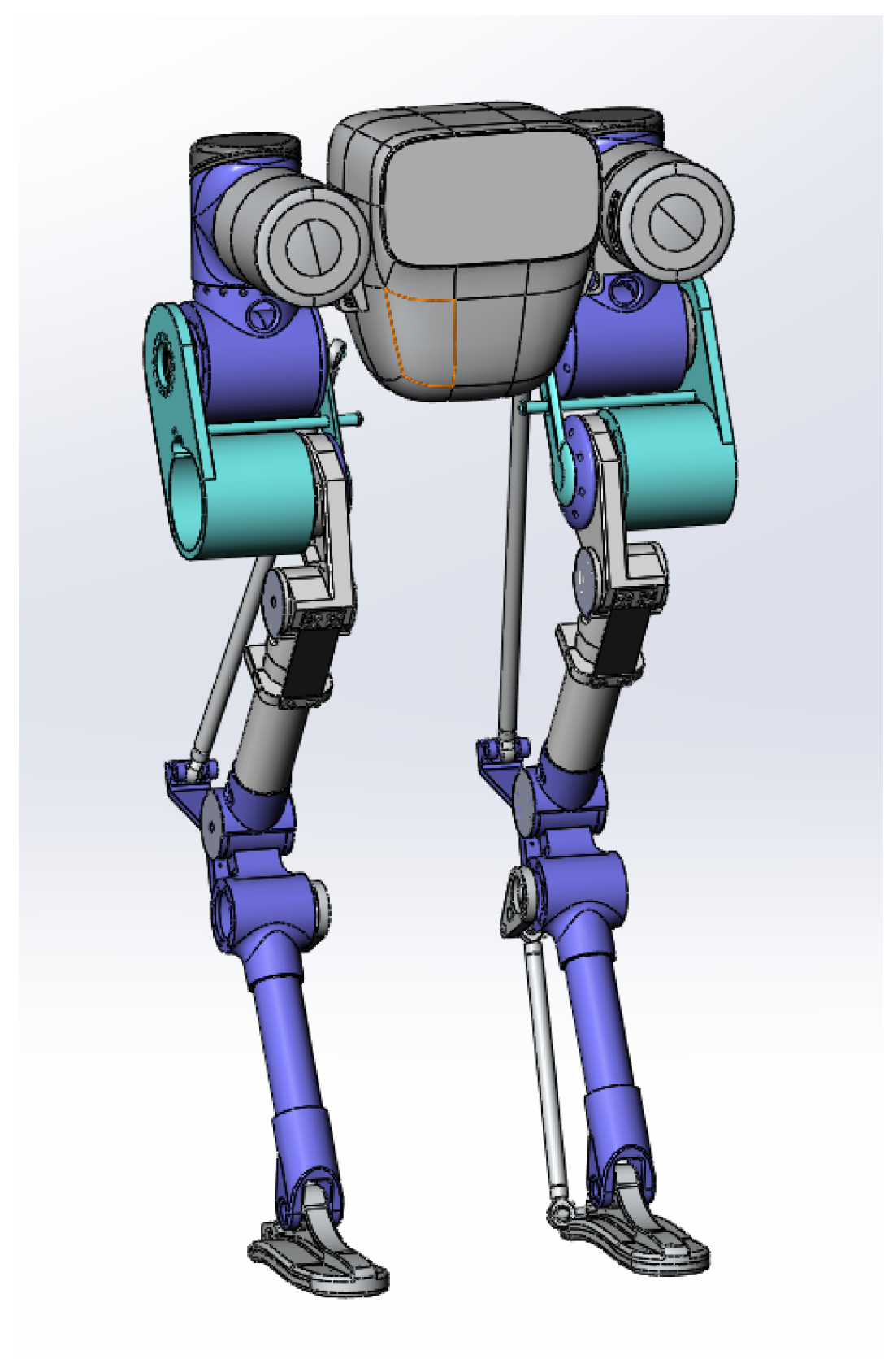This computer-generated image depicts a sophisticated robot with a predominantly gray-themed background, transitioning from light to darker grays in an ombre effect. The robot's design features intricate robotic legs that are a combination of blue, gray, and purple components. The feet are flat, chrome gray, and sturdy, providing stability. Ascending from the feet, the legs are segmented: the lower parts are blue, followed by gray actuators and joints that resemble metallic, hydraulic cylinders.

The legs connect to teal and purple sections, incorporating realistic-looking actuators and hydraulic pumps, creating a feasible design for practical usage. The joints and connections are highlighted with shades of teal and periwinkle blue, adding depth and technical detail. Notably, the upper sections include cylinder-like structures and flexing parts, simulating knee-like movements. 

The robot's upper body features a grayish head with a black, computer-screen-like face that includes round, blackish-gray elements on either side, resembling eyes or sensors, connected to a purple section. This section ties into the teal and gray components, ultimately attaching to the legs. The entire design is brought together with various screws and gears visible, adding to the realistic and functional appearance.